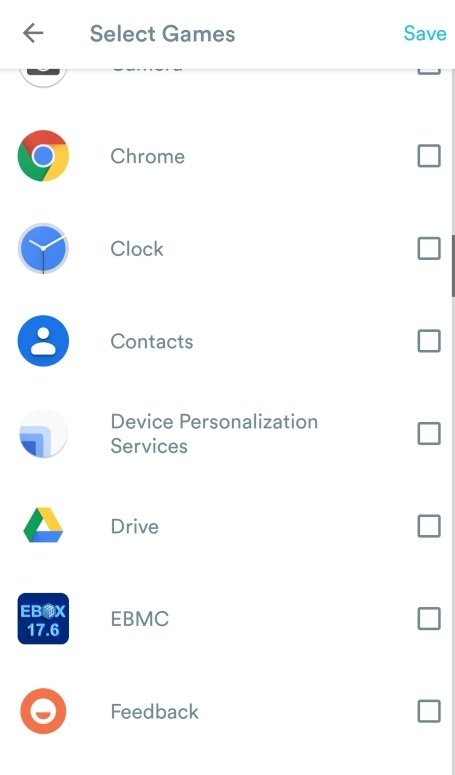In this screenshot of an Android device interface, the image showcases a selection screen for games. At the top left corner, there is a back button, and at the top right corner, a save button is visible. The display lists several apps: Chrome, Clock, Contacts, Device Personalization Services, Drive, EBMC, and Feedback. Each app listed includes a checkbox on its right side, and notably, none of these checkboxes have been selected or ticked.